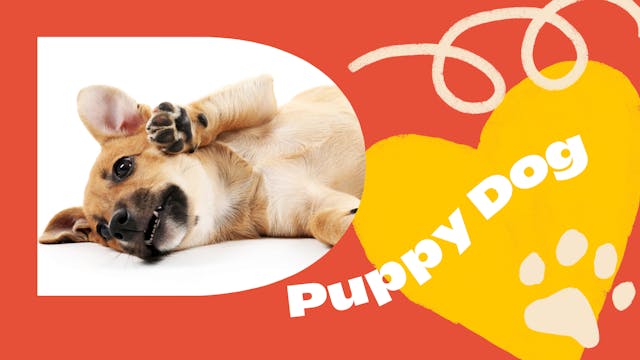This image features a light pink background with a gently curved, swirling white text that reads "puppy dog." Positioned to the left is a bullet-shaped frame with a white interior, containing an image of a small dog. The dog is orange and white, with black beady eyes, short ears, black paws, and a slightly blackened face with black hair around its mouth. It has light-colored fur on its chest and pink inside its ears. The dog is lying on its side, with one paw raised over its head, revealing its teeth slightly. A yellow heart near the right side of the image also contains the words "puppy dog" in white. Additionally, there's a light-colored squiggly line resembling a phone cord and a white paw print with four toes located in the bottom right corner.